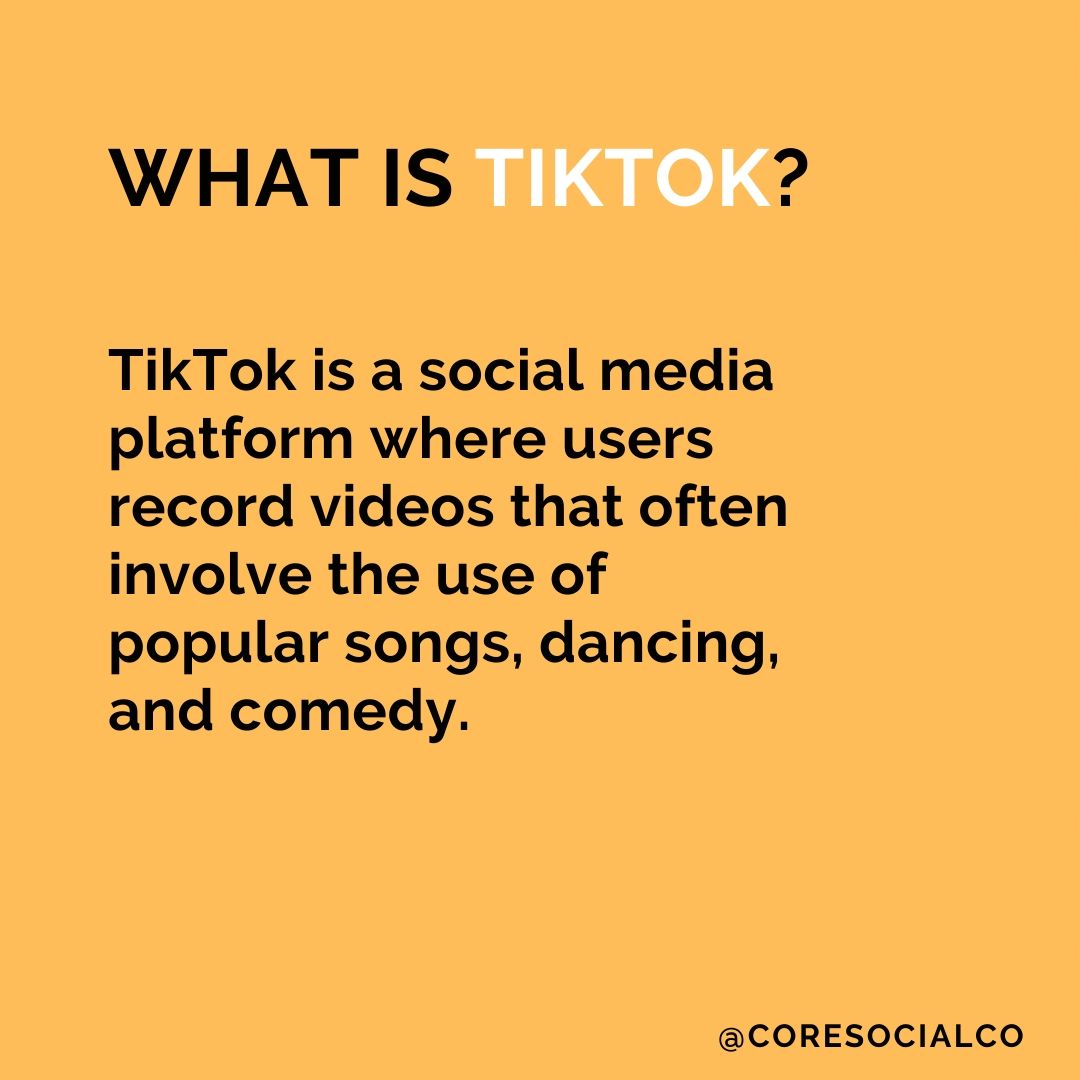**Detailed Caption:**

This image is a minimalist infographic with a yellow-gold background and black text, designed to provide a straightforward explanation of the social media platform TikTok. At the top of the image, there is a header with the question "What is TikTok?" prominently displayed, with the word "TikTok" highlighted in white text to stand out. The main body of the infographic describes TikTok as a social media platform where users record videos that often involve popular songs, dancing, and comedy. This content appears to be aimed at individuals who may not be familiar with the platform, possibly an older audience or parents of young children who might be using TikTok. The text is positioned towards the top left of the image and is relatively large for ease of reading. A credit is given to "@coresocialco" at the bottom right corner, indicating the creator or source of the infographic. The overall design is very simple and clean, making the information easy to comprehend at a glance. This graphic was likely shared on another social media platform such as Twitter or Instagram, to educate and inform users.